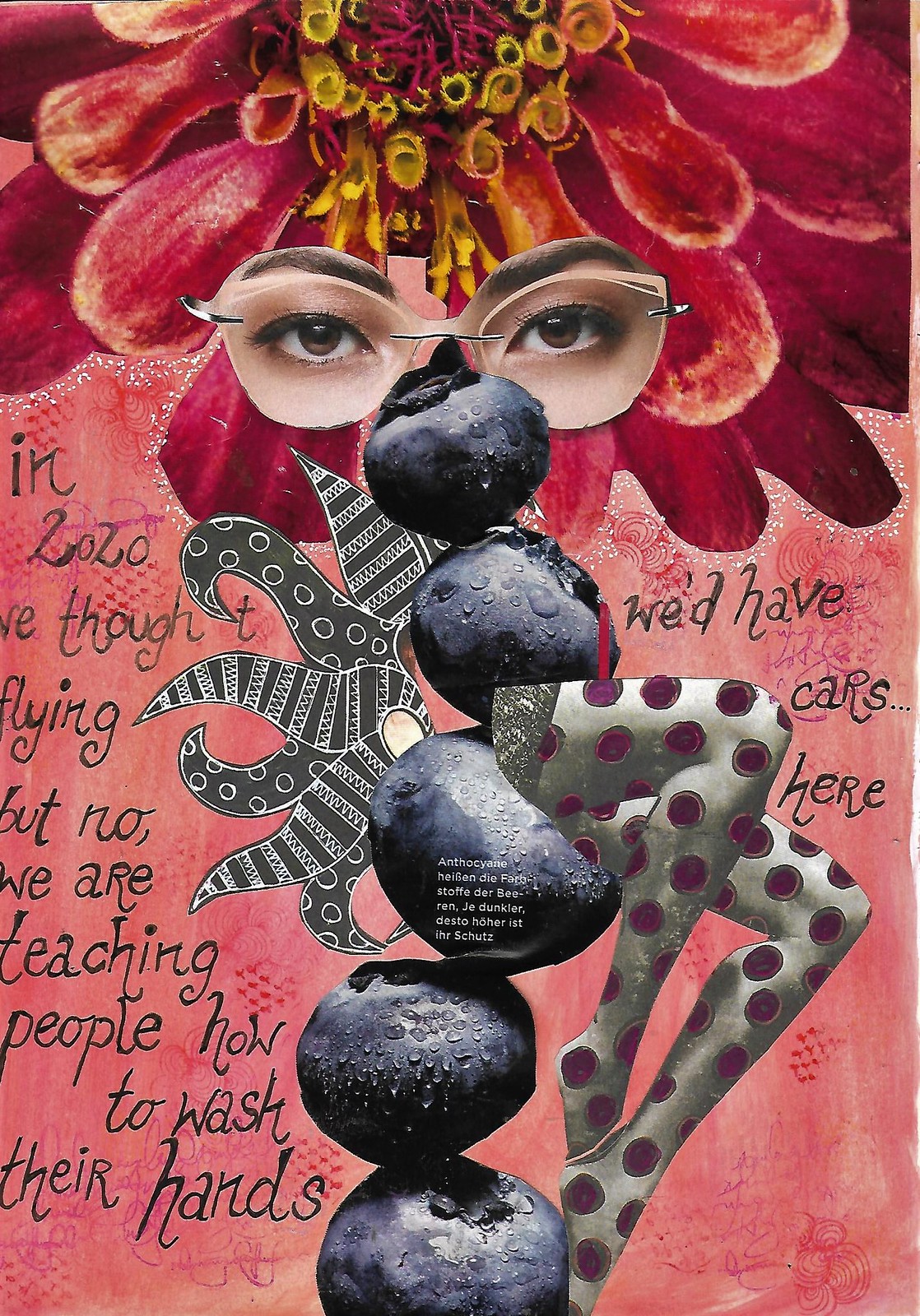The image is a detailed and eclectic collage. At the top, there is a prominent red flower with numerous petals and yellow filaments protruding from its center, which may resemble a rose or zinnia. Below this flower, a pair of realistic-looking eyes, set behind glasses, peep out with black eyebrows and dark brown irises. Surrounding the eyes is a pink-hued background. Below the eyes, a vertical alignment features five blueberries. Between the second and third blueberries, there is a pair of women’s legs, oriented to the right, wearing pants adorned with large purple round patterns. To the left side of the stones, what seem to be tentacles are visible. Scattered throughout the image, there is handwritten text, stating, "In 2020 we thought we'd have flying cars but now we are teaching people how to wash their hands" and "We would have cars here." This varied and whimsical composition blends natural elements with human features and abstract designs.